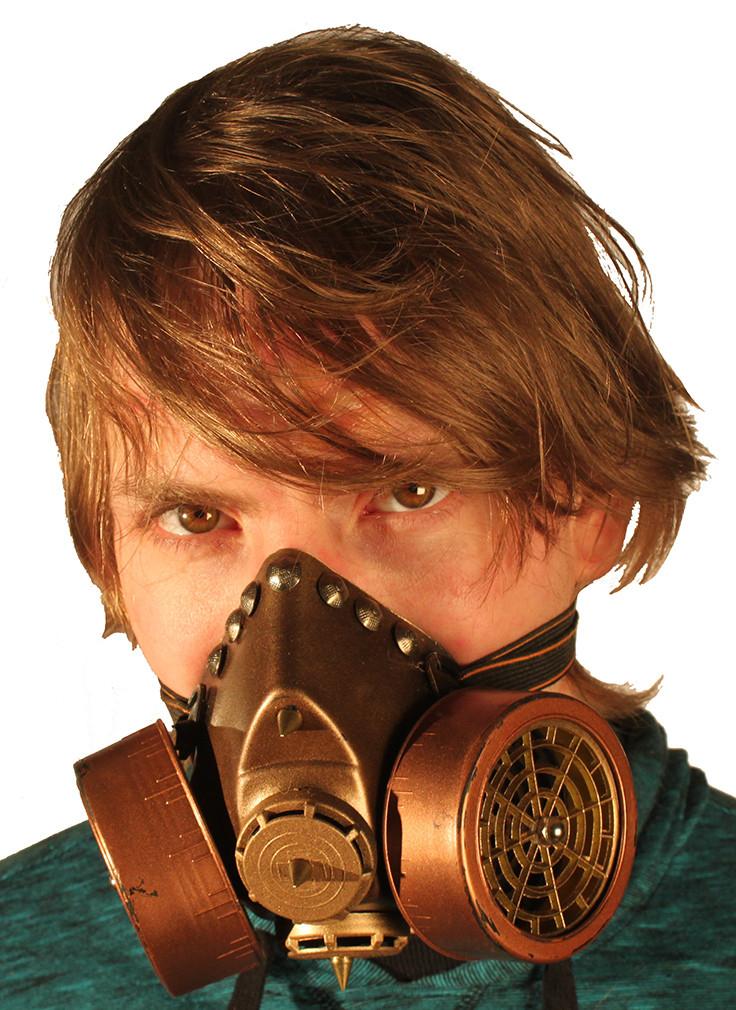A Caucasian man is depicted wearing an antique gas mask. He has light brown hair, parted on the left side and combed across to the right, reaching down to his ears. His brown eyes stare straight forward behind the mask, which has a distinct metal copper color. The mask features tiny silver circles along the top of the nose piece, and a prominent circular section with a point at the end at the front and bottom. On both sides of the mask, there are darker colored circles resembling ventilation filters, each detailed with lines and a central circle. The mask is secured with a black strap, accented with orange lines at the top and bottom, that wraps tightly around the man’s neck. The man is dressed in a shirt that mixes light and dark teal shades, which might be a hoodie. However, there's visible photo editing under his right ear, where the background shows jagged edges.